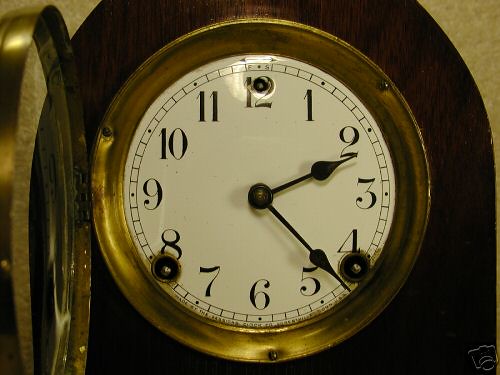This detailed photograph features an antique-style clock, reminiscent of a grandfather clock. The clock is encased in a wooden structure with an ornate brass bezel surrounding its face. Its glass cover, designed to open outward on a hinge, is currently swung open to the left. The clock’s face is a beige to off-white color, displaying black numerals in a traditional sequence from 1 to 12, with black metal hands pointing at 2:23 p.m.

The face is further characterized by three winding gears positioned at 12, 4, and 8 o'clock, each marked by golden areas, thought to be screws. Notably, the number 12 has a puncture hole, adding to its vintage charm. The entire setting is illuminated from the front, casting a reflective glow near the top of the clock face. The clock is mounted against what seems to be a sandstone-colored wall, which adds a warm backdrop to the overall composition. In the lower right corner of the clock face, there is a subtle watermark depicting a pig's head, rendered in a transparent white sketch. The main focus of the photograph is the strikingly detailed clock face, dominating the image and encapsulating the timeless elegance of its antique design.